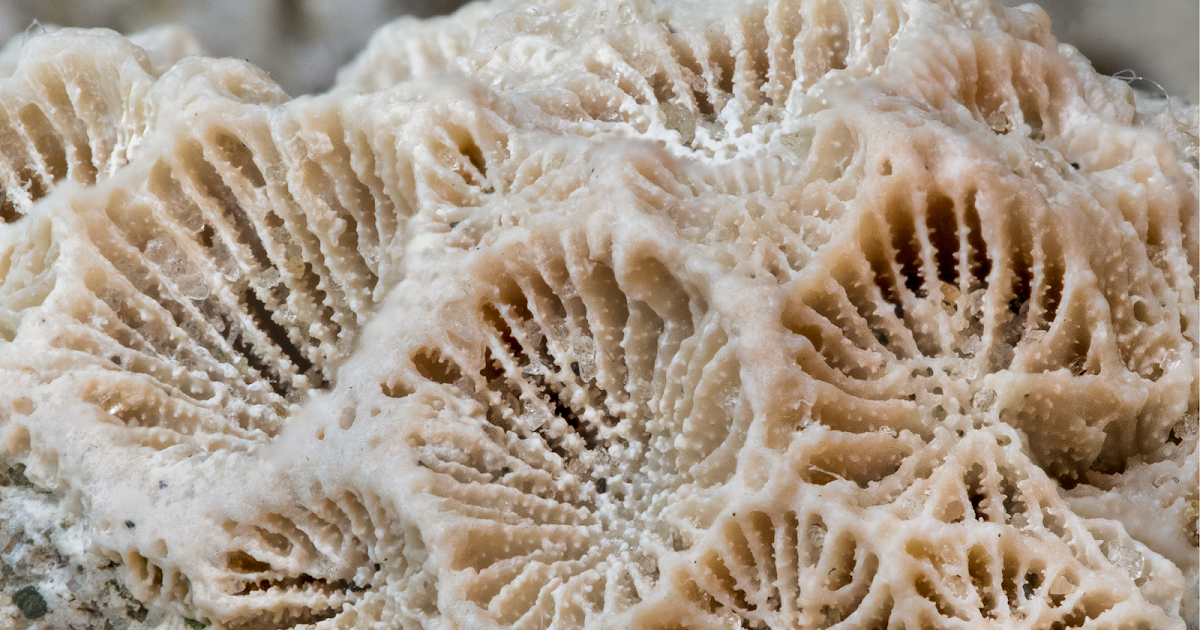This image depicts an underwater structure resembling coral, characterized by a central white formation with small divots and radial, carved lines. The structure has a mound-like overall shape and appears light golden-brown or tan in color. These formations, resembling imprints or designs found on shells, display rocky, solid patterns and branching structures that extend outward from the center, giving them a circular, wheel-like appearance. The intricate detailing suggests a close-up of an organism or formation typically found in deep-sea environments.